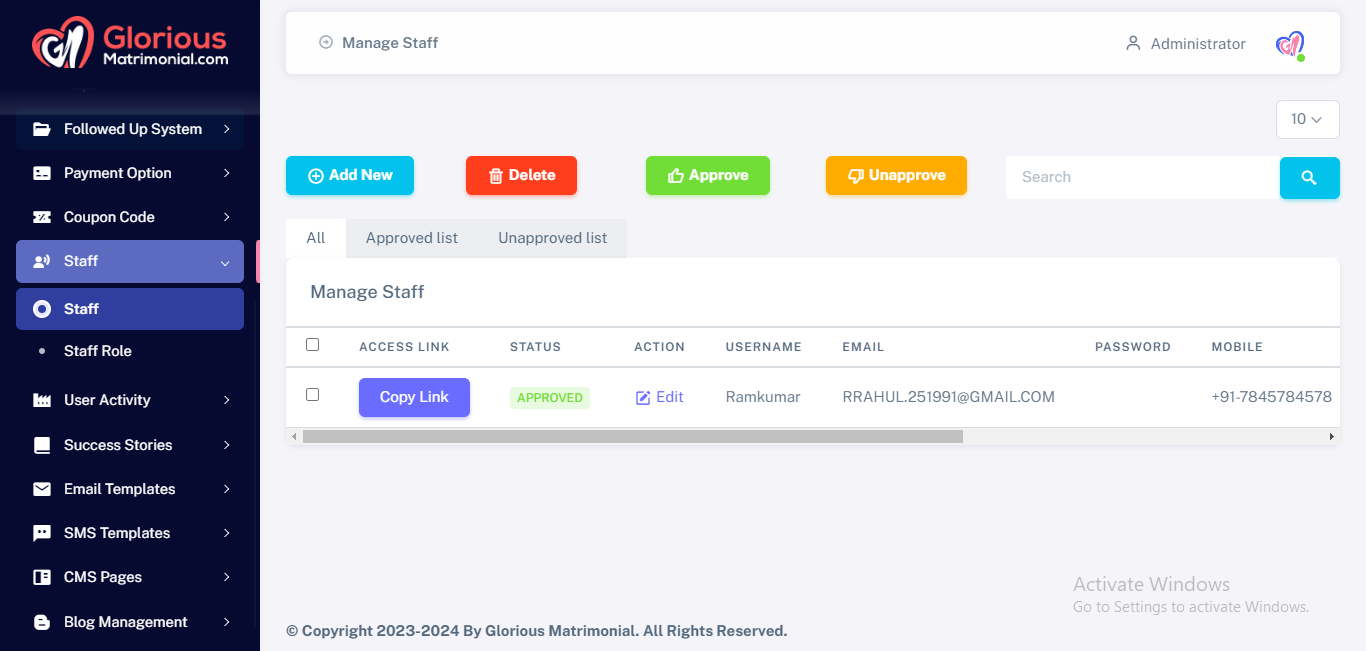Here's a detailed and cleaned-up caption for the screenshot:

---

This screenshot captures a webpage from GloriousMatrimonial.com. The left column of the page features a navigation menu set against a dark blue background. At the very top left, a prominent red heart-shaped icon is displayed, accompanied by the website's name: "Glorious" in red text followed by "Matrimonial.com" in white text.

The vertical navigation menu includes multiple options: 
- Follow-Up System
- Payment Option
- Coupon Code
- Staff
- Staff Role
- User Activity
- Success Stories
- Email Templates
- SMS Templates
- CMS Pages
- Blog Management

The "Staff" and "Staff Role" options in the menu are highlighted in blue, indicating their active status.

On the right side of the page is the staff management section. It provides various fields and options for managing staff members, including: 
- Administrator Sign-In
- Access Link
- Status
- Action
- Username
- Email
- Password
- Mobile